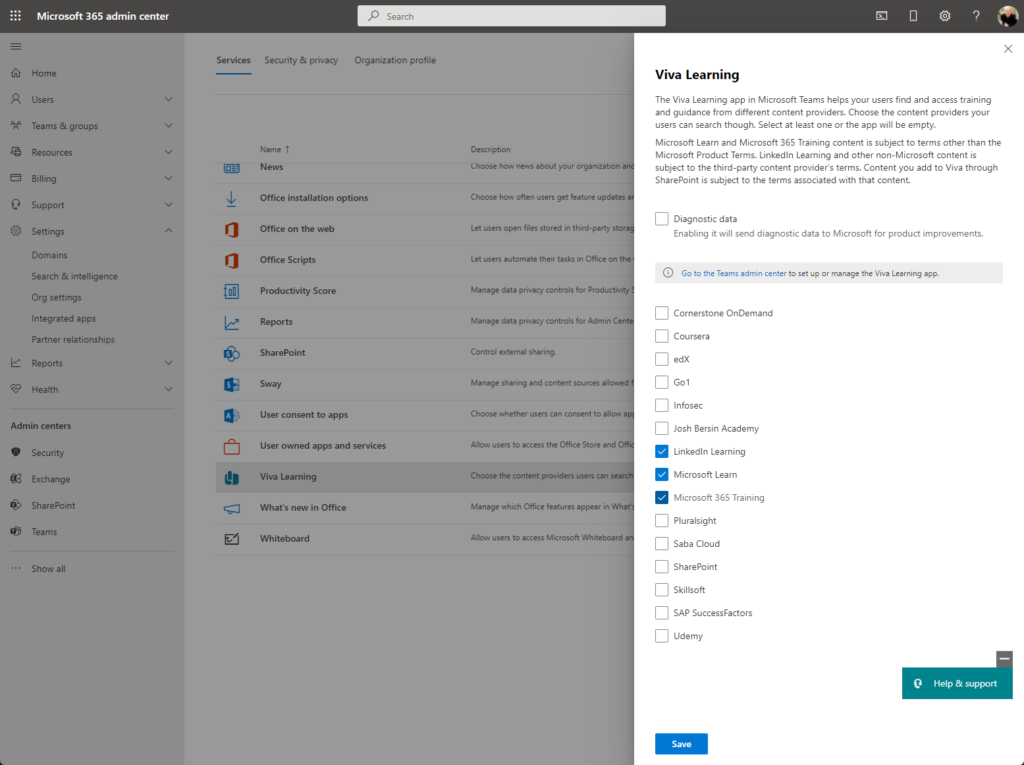This screenshot showcases the Microsoft 365 Admin Center with a right-side tab open, causing the rest of the interface to be grayed out but still visible. The highlighted tab is titled "Viva Learning."

In this detailed view, a paragraph explains that the Viva Learning app within Microsoft Teams assists users in finding and accessing training and guidance from various content providers. Admins are prompted to select at least one content provider to enable search functionality within the app; otherwise, the app appears empty. Important distinctions about content limitations and terms are made:
- Microsoft Learn and Microsoft 365 training content adhere to specific terms distinct from the general Microsoft product teams.
- Content from LinkedIn Learning and other non-Microsoft providers follows third-party content provider terms.
- Any content added to Viva through SharePoint must comply with the terms linked to that content.

Beneath this explanation, there is a checkbox related to diagnostic data that, when enabled, sends diagnostic information to Microsoft to aid in product improvements.

A comprehensive list of content providers is presented with checkboxes next to each option, including:
- Cornerstone OnDemand
- Coursera
- edX
- Go1
- InfoSec
- Josh Bersin Academy
- LinkedIn Learning (selected)
- Microsoft Learn
- Microsoft 365 Training (selected)
- Pluralsight
- Saba Cloud
- SharePoint
- Skillsoft
- SAP SuccessFactors
- Udemy

In this instance, LinkedIn Learning, Microsoft Teams, and Microsoft 365 Training are already selected.

Everything else in the screenshot, such as the main application interface, remains visible albeit grayed out due to the active sidebar. The user focus is clearly directed to configuring the Viva Learning app settings and content provider selections for an optimized training experience within Microsoft Teams.